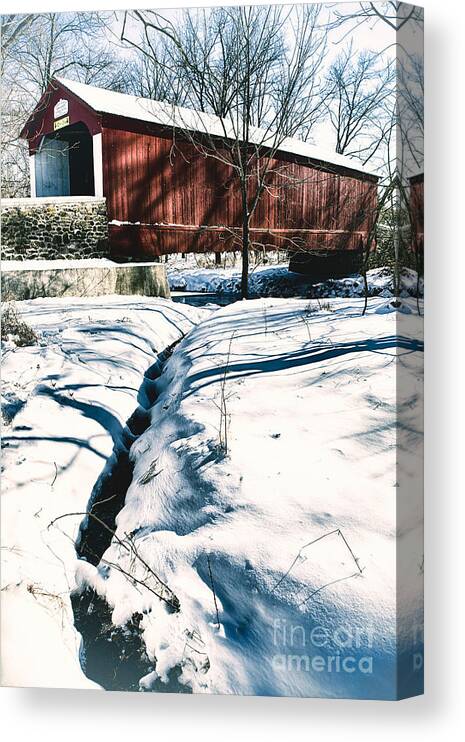This image features a detailed photograph printed on canvas, available for purchase on a website, with a prominent Fine Art America watermark in the bottom right corner. The scene captures a wintry landscape characterized by a snow-covered ground and barren trees devoid of leaves, emphasizing the desolate beauty of the season. Central to the image is an old, wooden structure that resembles a tunnel or covered bridge, painted in a reddish hue with dark brown and white wooden elements. The structure is flanked by gray stone walls leading up to it, suggesting a rural or countryside setting. The backdrop includes a subtle indentation in the snow that indicates a potential stream running through the area. The entire scene exudes a serene, almost monochromatic palette dominated by whites, grays, and browns, highlighting the quiet stillness of winter.